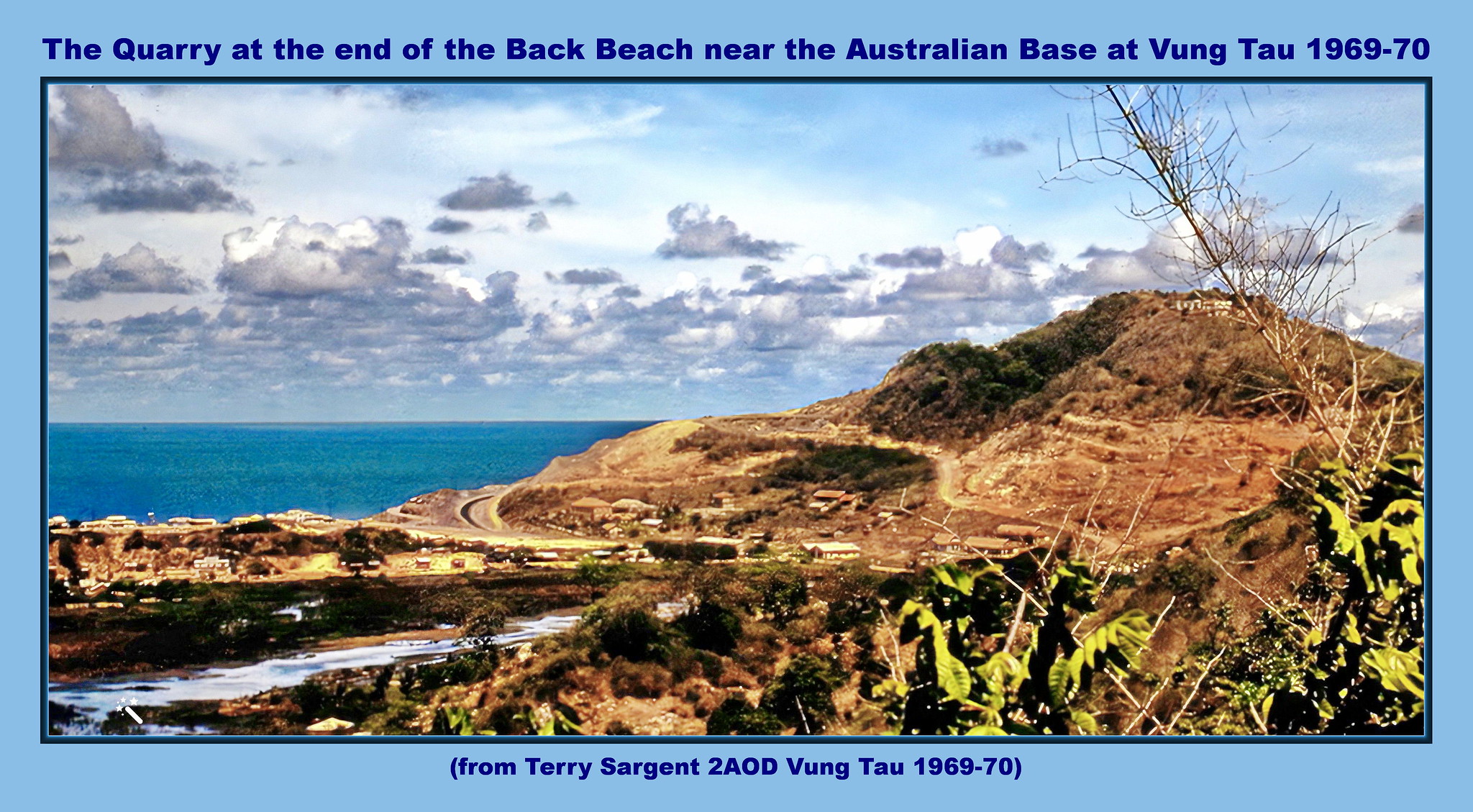This image, designed like a postcard, showcases the quarry at the end of Jack Beach near the Australian base at Vung Tau during 1969-1970. The scene captures a serene beach with blue water extending from the left to the center, partially obscured by a slightly elevated brown dirt hill on the right. Puffy gray and white clouds hover over the landscape, contrasting against the blue sky primarily in the upper right corner. The foreground features a road winding past simple, hastily crafted Southeast Asian structures and dead vegetation, including a prominent leafless tree. The bottom of the image reads "From Terry Sergeant, 2AOD Vung Tau, 1969 to 70," grounding the scene in its historical context.